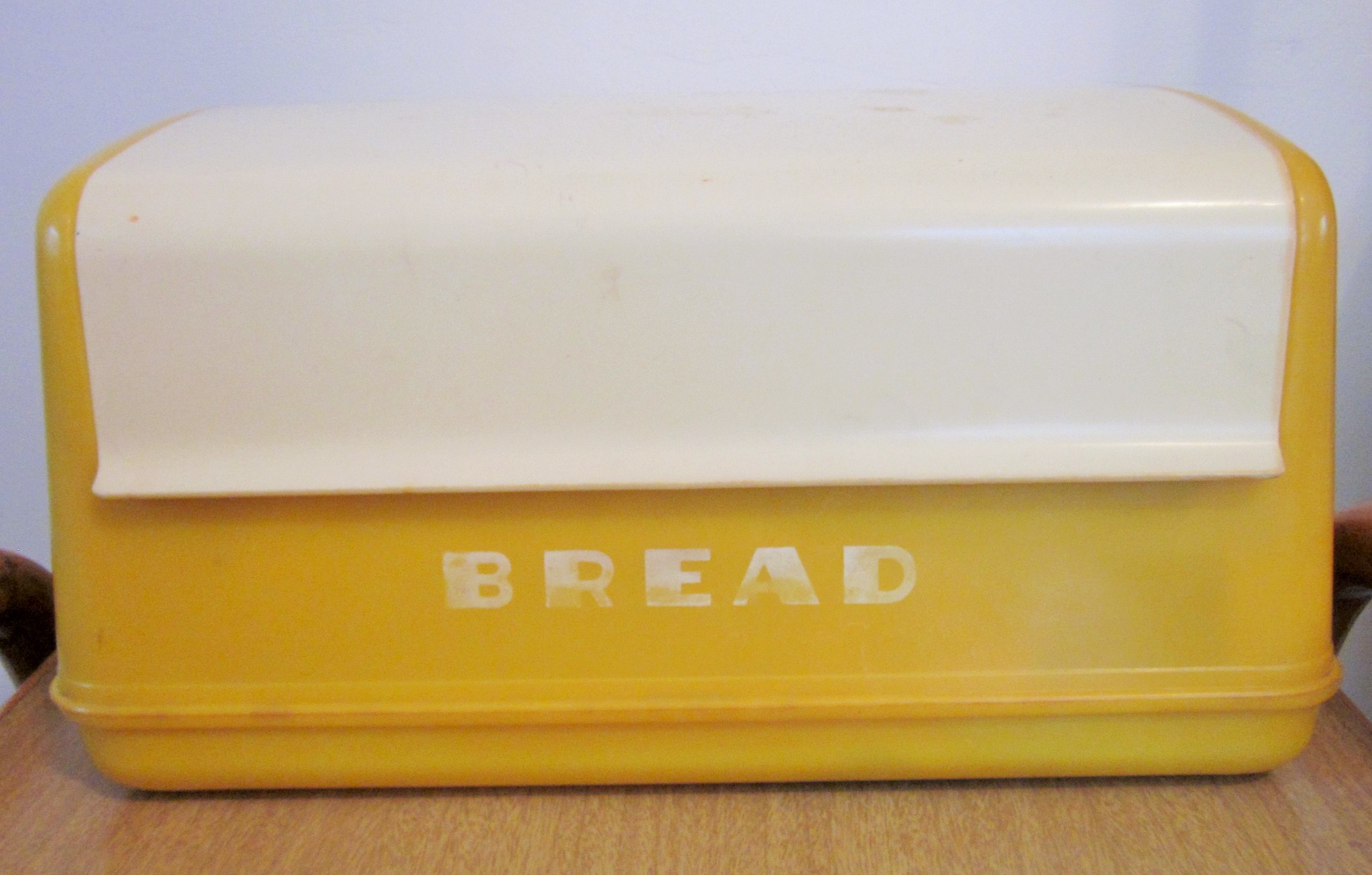This image features a vintage, yellow plastic bread box sitting atop a wooden push cart. The bread box has a white plastic lid, which is slightly worn and stained, typical of a vintage item. The word "BREAD" is displayed in capital letters on the front of the box, written in a white font that is faded and worn. The lid does not extend all the way to the edges and features a small lip, presumably acting as a handle for lifting. The bread box is relatively small, capturing the feel of a makeup tote in terms of size. The wooden push cart has reddish handles visible on both sides. The background of the image shows a wall in a whitish blue hue, contributing to the overall aged and nostalgic feel of the scene.